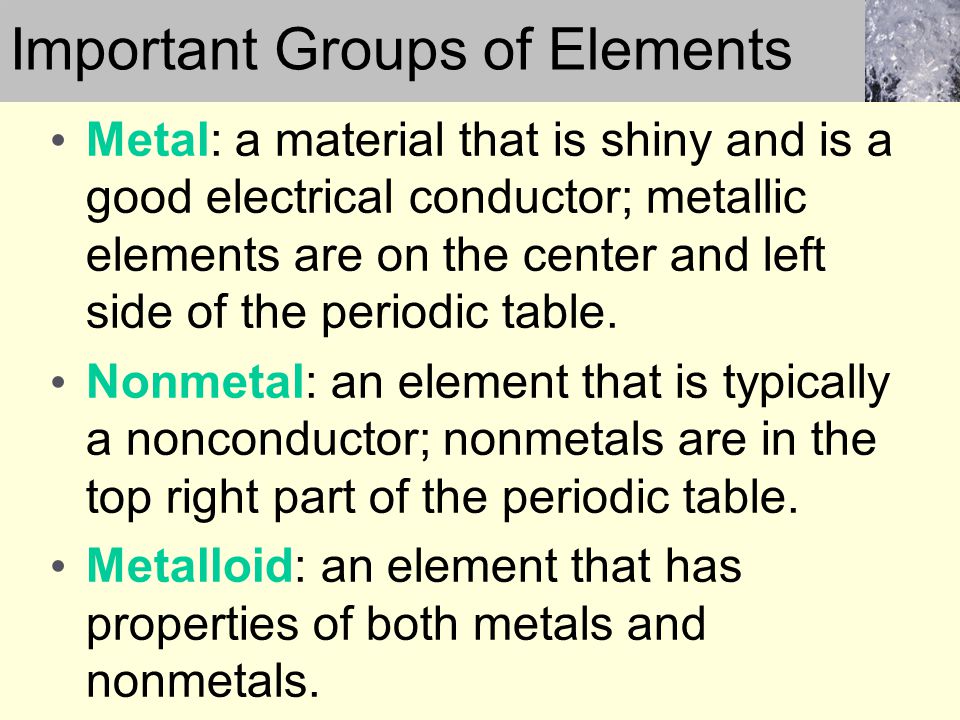The image appears to be an educational PowerPoint slide titled "Important Groups of Elements" displayed in black text on a gray background. In the top right corner, there's a small, somewhat unclear image that looks glassy or like water. The main section of the slide has a light tan or yellow background featuring three black bullet points with headings in green or cyan blue. The three bullet points describe different classes of elements: 

1. **Metal**: Defined as a material that is shiny and a good electrical conductor, with metallic elements situated on the left and center of the periodic table.
2. **Nonmetal**: Described as an element that is typically a non-conductor, with nonmetals located in the top right part of the periodic table.
3. **Metalloid**: Explained as an element that has properties of both metals and nonmetals.

The slide is likely designed for an educational setting, possibly for use in a classroom.